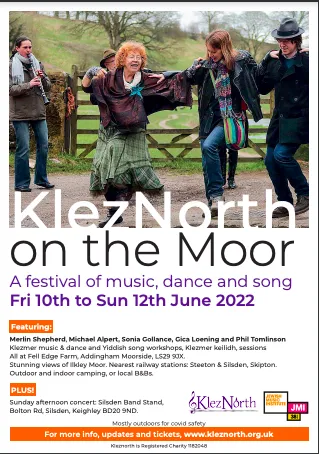The poster for Klez North on the Moor Music Festival showcases a vibrant outdoor scene of five Caucasian individuals engaged in lively line dancing. Positioned in a circle with arms interlinked and joyous expressions, the dancers include an older woman on the left and younger participants in their 20s and 30s. A clarinet player enhances the festive atmosphere. The setting is a fenced-in area on a hillside adorned with trees, everyone dressed warmly in jackets. The event, scheduled from Friday, June 10th to Sunday, June 12th, 2022, promises music, dance, and song with performances from Marilyn Shepard, Michael Alpert, Sonja Gollins, Zika Zoning, and Phil Tomlinson. The design of the flyer features a prominent photo of the dance scene at the top with white and purple text detailing the festival against a white background. Key information, including a mention of COVID safety measures and additional concert details, is highlighted in an orange banner at the bottom. For more updates and ticketing info, the website kleznorth.org.uk is provided. The bottom right corner contains logos of supporting businesses and the town.